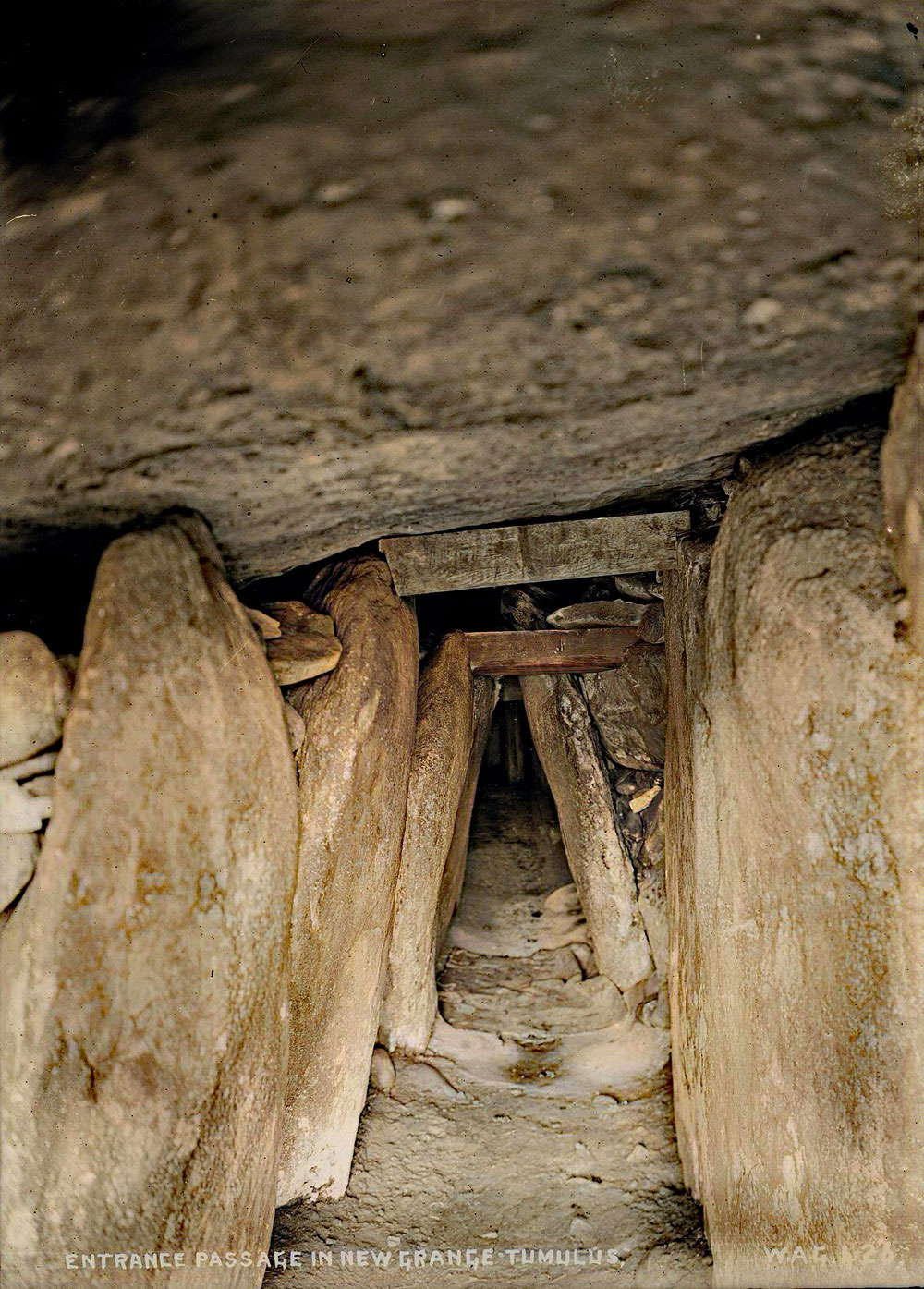The image depicts the Entrance Passage in the New Grange Tumulus, displaying an ancient tunnel made up of large, tan and gray stones arranged in a triangular formation. The weathered and dirty rocks, some possibly granite, form the walls and ceiling of the passage. The construction includes a narrow top and wider base, with additional wooden bracing connecting the stones. The sandy and rocky floor is strewn with dirt and shows some evidence of steps that have traversed through the corridor. As the passage extends, it fades into darkness, accentuating the eerie, shadowy atmosphere. A watermark at the bottom of the image reads “Entrance Passage in New Grange Tumulus,” accompanied by some indistinct markings, possibly “WAG Something 23.”